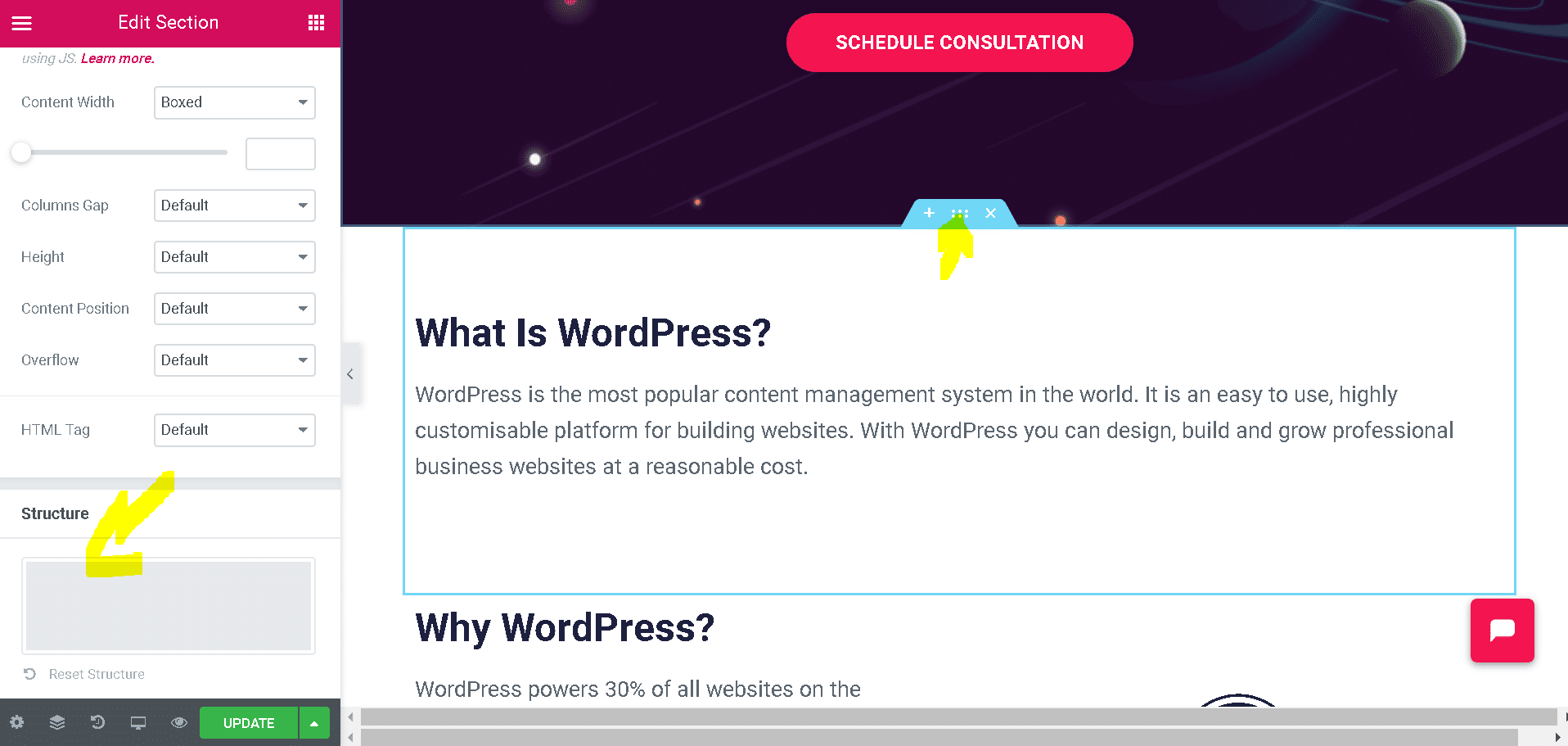The image displays a user interface of someone creating their WordPress website. Central to the image is a blue box containing the text:

"What is WordPress?
WordPress is the most popular content management system in the world. It is an easy to use, highly customizable platform for building websites. With WordPress, you can design, build, and grow professional business websites at a reasonable cost."

A yellow arrow originates from this blue box, pointing upwards towards a gray box labeled "edit section." This section, positioned on the left-hand side in a reddish area, includes various setting fields: "Content Width Boxed," "Columns Gap Default," "Height Default," "Content Position Default," "Overflow Default," and “HTML Tag Default." Beneath these fields, it reads "Structure."

In the lower part of the image, there is a darker area with multiple symbols, culminating at the right with a green button labeled "Update."

On the right side, above the WordPress description, there is a background image depicting outer space, featuring stars and a planet. A red button labeled "Schedule Consultation" is visible at the top of this section. At the bottom of the interface, there’s a partial text that reads, "Why WordPress? WordPress powers 30% of all websites on the…" and then cuts off.